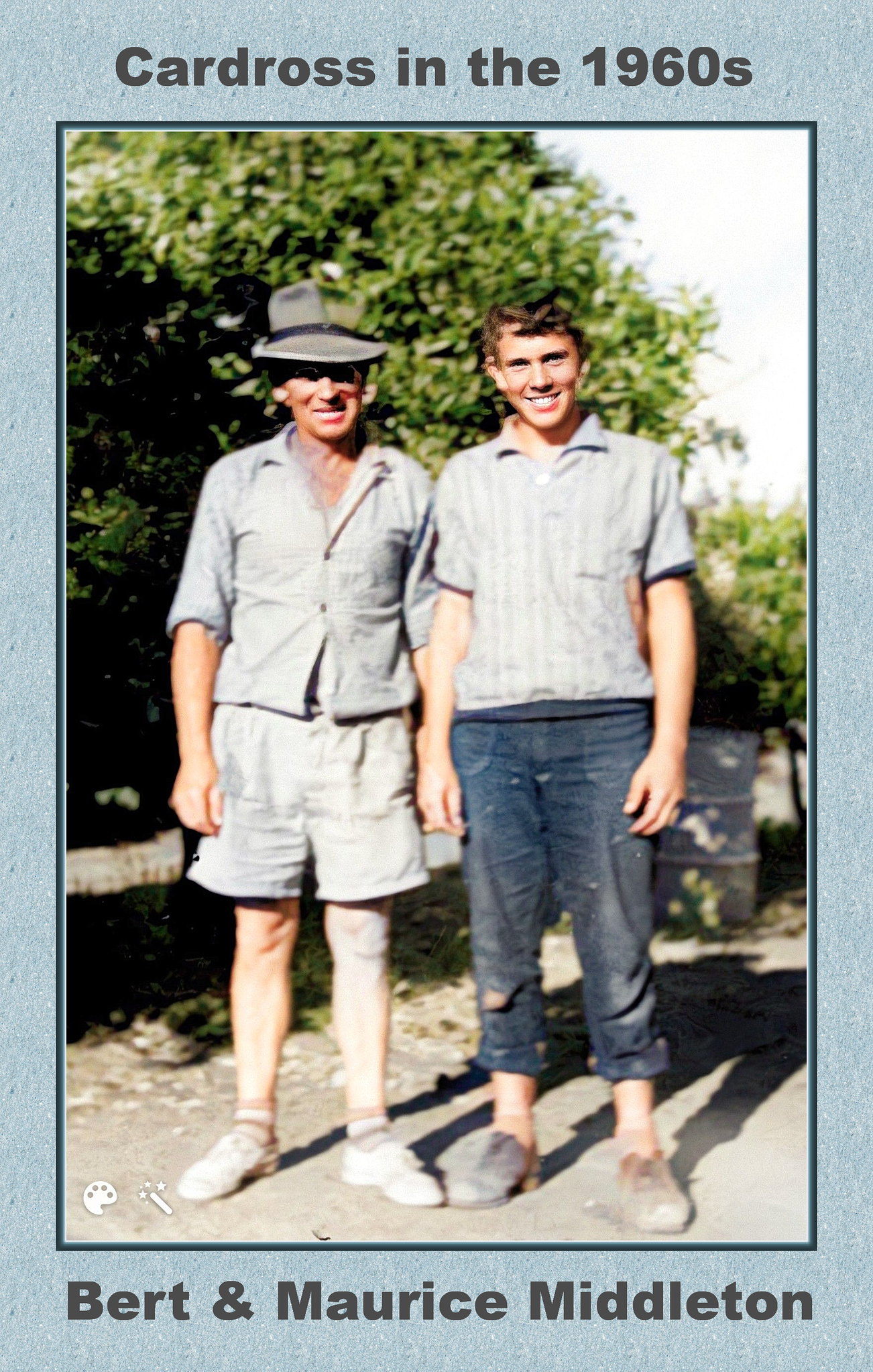This is an older, vertical photograph from the 1960s, bordered by a light blue frame with dark gray captions. At the top, it reads "Card Ross in the 1960s," and at the bottom, "Burt and Maurice Middleton." The image features two smiling men standing side by side on a sunlit cement surface. The man on the left appears older, possibly in his 30s or 40s. He is dressed in a gray fedora, a gray button-up shirt, gray shorts, white shoes, and ankle socks. His hair is hidden under his hat. The man on the right seems younger, likely in his late teens or early 20s, with dark brown hair. He is wearing a light blue short-sleeved collared shirt, blue jeans rolled up at the ankles, and dusty dark brown shoes. Both men are clean-shaven. The background showcases a lush, green area with large trees. On the right side of the image, behind the younger man, there is a gray garbage can. The sunlight creates long shadows behind them, indicating it is daytime.